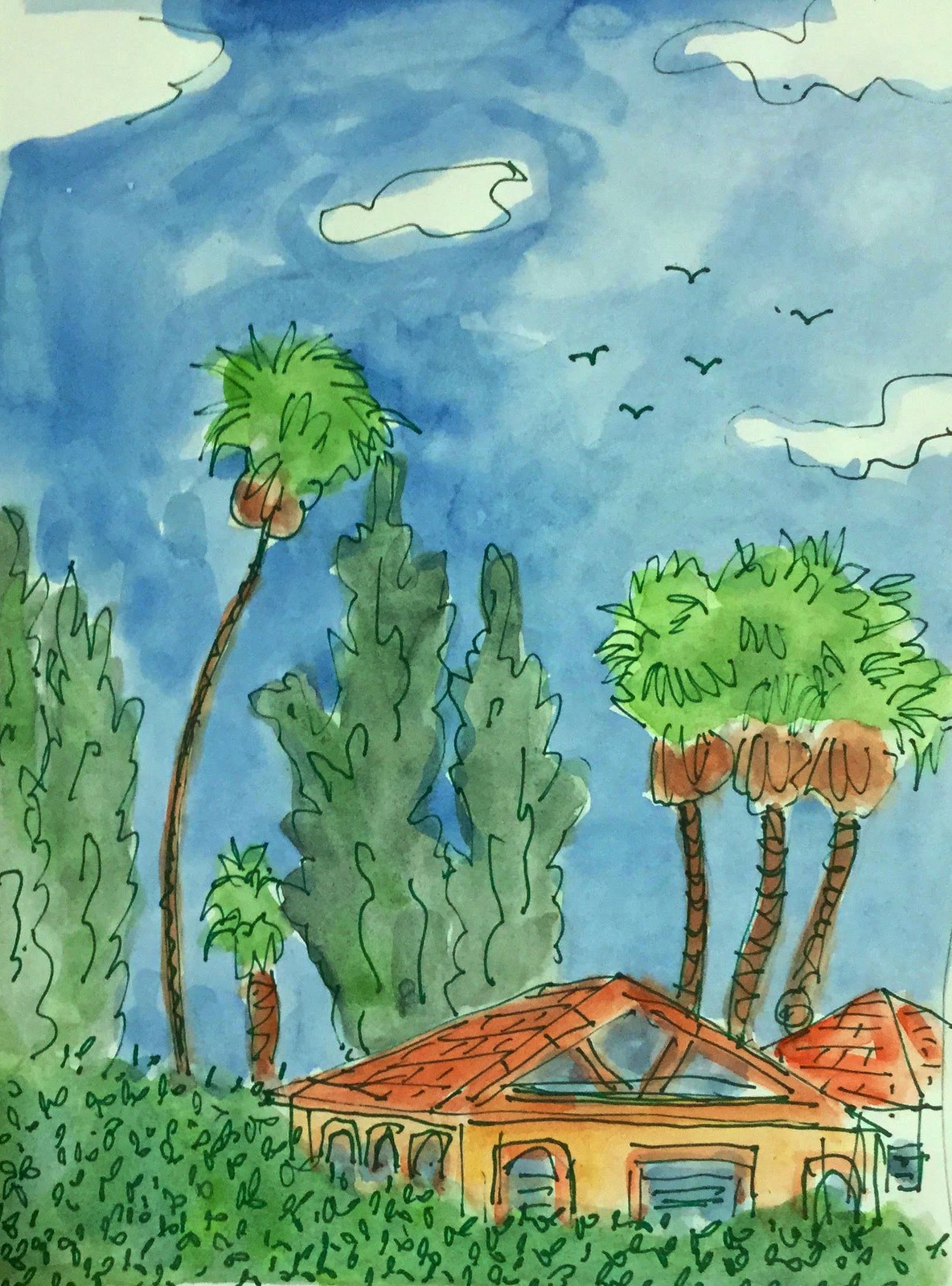The image is a vertically aligned, portrait-mode watercolor drawing depicting a tropical scene. At the forefront, a neat home with a reddish-brown tiled roof and a skylight window sits nestled among tall palm trees and other taller trees. The house itself has a tan-yellowy facade with three windows on the side, two windows at the front, and a front door, partly obscured by grass growing in the foreground. To the right of this main house is another structure with a similar reddish-brown roof but a white exterior, decked with a small window. Blue skies with scattered clouds form the backdrop, adorned with a flock of five birds flying above. The landscape features a large bush in the front, along with various grasses, adding to the serene, tropical ambiance.